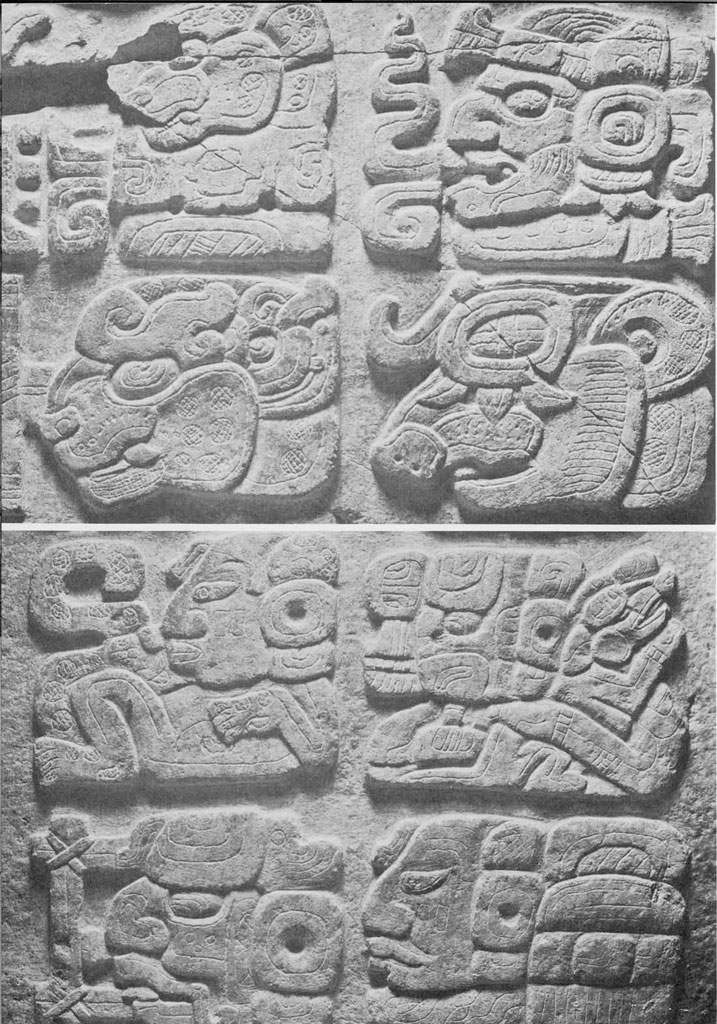The black and white photograph prominently features two rows of ancient stone carvings, with eight intricately detailed figures in total—four in the top row and four in the bottom. Each carving is set in a stone wall and faces to the left, exuding an aura of antiquity, possibly from the Mayan era. In the upper left, the stone is cracked, revealing a triangular break and cloud-like swirls. Next to it, a carving depicts an animal with long hair, while another showcases a warrior-like figure adorned with headwear. The final figure in the top row appears to be turtle-shaped. The bottom row presents an array of similar artistic prowess, featuring a lion and a bull on the left and right respectively. In between, a monkey and a dragon join a man and a partially hidden male figure behind a pillar, further emphasizing the historical essence of the tableau. This striking image captures these timeless stone carvings, offering a fascinating glimpse into ancient artistry.